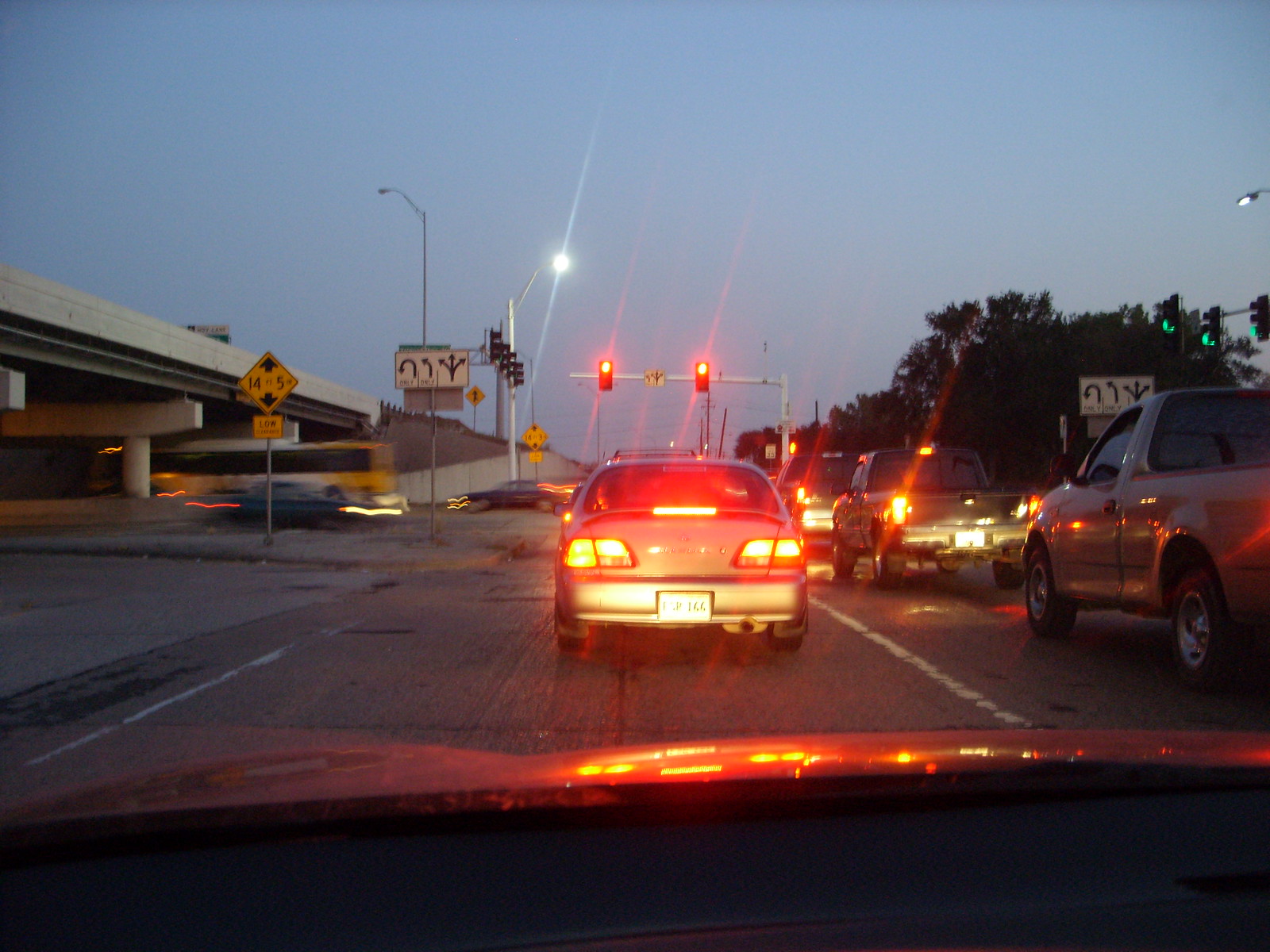The photograph captures an outdoor twilight scene taken from within a vehicle, through the windshield, at an intersection waiting to merge onto a freeway. The sky is a dark blue, and the ambient light combines with vehicle headlights to create a dimly lit atmosphere. The image shows two rows of cars, many with illuminated brake lights, stopped at a red signal. Among the vehicles is a large white bus with yellow accents and tinted windows traveling on the freeway. On the left side of the image, there is an overpass supported by large concrete pillars, with a clearly visible yellow and black clearance sign reading "14-5" indicating 14 feet and 5 inches. To the right, a group of trees lines the road. The road signs indicate lane directions while red streetlights and the reflection from the car ahead add to the composition. The front part of the vehicle being driven is visible with reflections on the hood from the red traffic light, adding a dynamic quality to the scene. Trees are visible on the right-hand side, adding to the complexity and depth of the photograph.